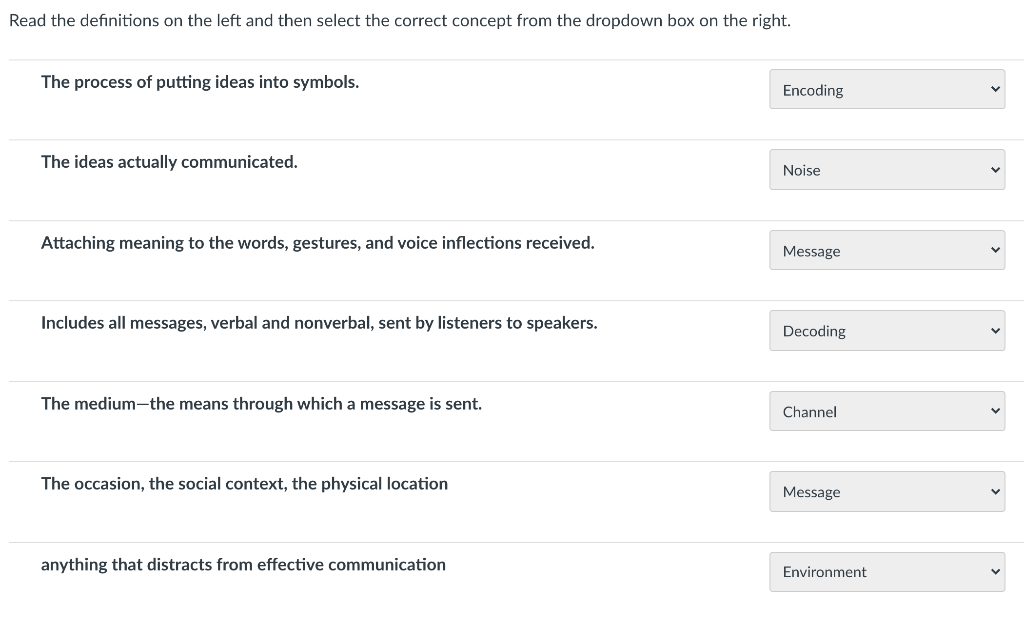The image features a vertical layout with a white background and a clear instructional prompt at the top. The prompt, written in black font, reads: "Read the definitions on the left and then select the correct concept from the drop-down box on the right." Below the prompt, several terms and their corresponding definitions are organized within boxes separated by horizontal light gray lines.

1. The first box contains the definition "The process of putting ideas into symbols," with the bolded black word "encoding" in a horizontal rectangular light gray box on the right. The right side of this box displays a small downward arrow in black.
2. The second box presents the definition "The ideas actually communicated," accompanied by the word "noise" in a similar format on the right.
3. The third box defines "Attaching meaning to the words, gestures, and voice inflections received," with the word "message" on the right.
4. The fourth definition is "Includes all messages, verbal and nonverbal, sent by listeners to speakers," and the right side features the word "decoding."
5. The fifth definition provided is "The medium – the means through which a message is sent," with "channel" appearing on the right.
6. In the sixth box, the definition "The occasion, the social context, the physical location" appears on the left, with "message" on the right.
7. Lastly, the definition "Anything that distracts from effective communication" is paired with the word "environment" on the right.

Each entry on the left side is bolded in black, corresponding to the text inside the light gray boxes with downward arrows on the right, indicating a drop-down selection feature.